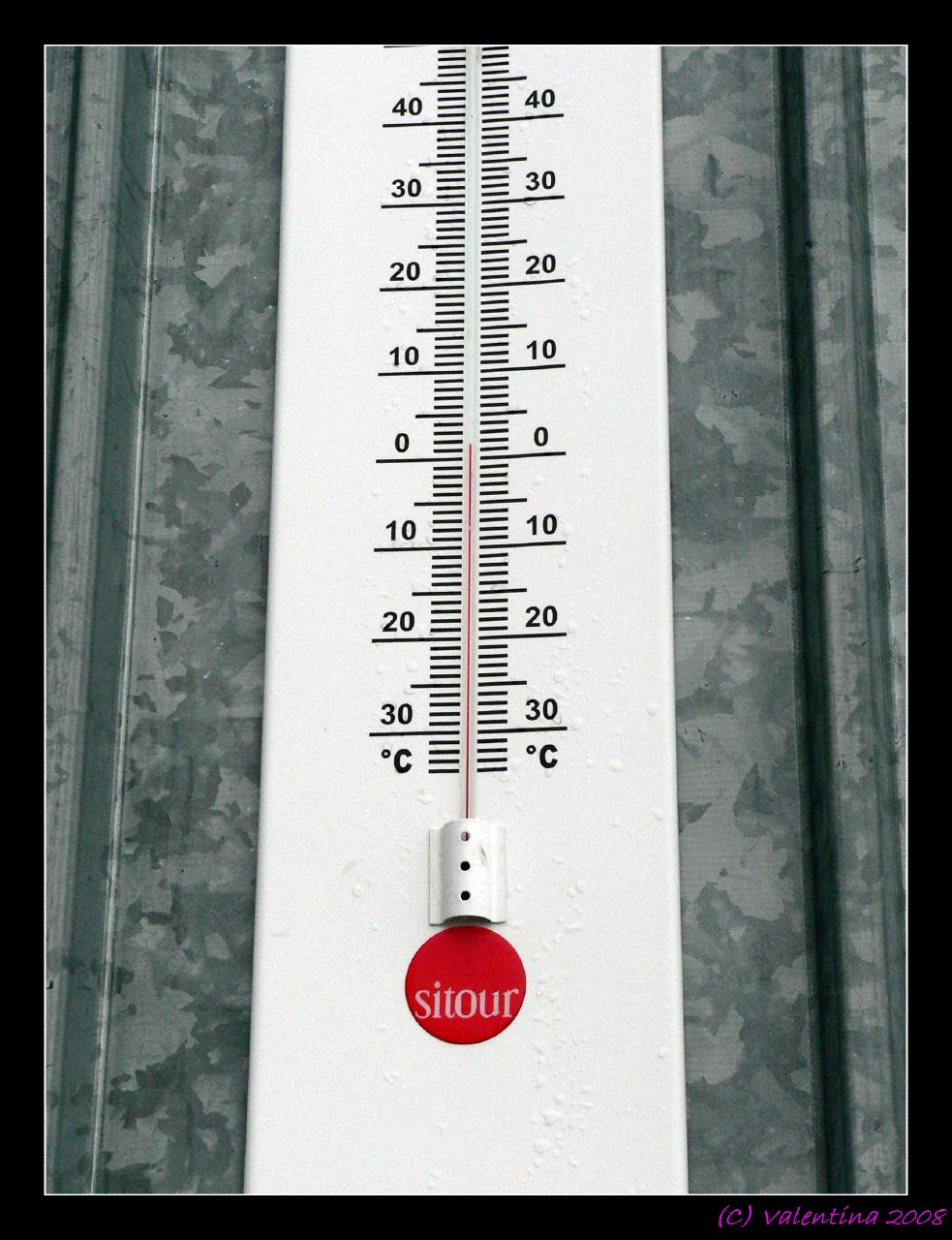This image features a vintage, black and white thermometer prominently displaying temperatures in Celsius. The thermometer, labeled with the brand name "S-I-T-O-U-R," contains a striking red marking at the bottom designed to mimic mercury. The top part of the thermometer is cropped out of the frame, adding a sense of focus to its details. 

Mounted against a gray, marbled surface that appears to be part of a wall, the setting includes paneling on either side potentially framing a door or window, suggesting an indoor environment. The photograph is bordered by a thick black edge with a thinner white border inside, giving it a refined presentation. There is noticeable paint bump texture on the thermometer, contributing to its aged, possibly antique aesthetic.

At the bottom right corner of the image, a photo credit is clearly visible, stating "© Valentina 2008," verifying the authenticity and ownership of the photograph. Despite the simplicity of the subject, the image captivates with its rich textures and meticulous composition, allowing a glimpse into a functional yet aesthetically pleasing piece.